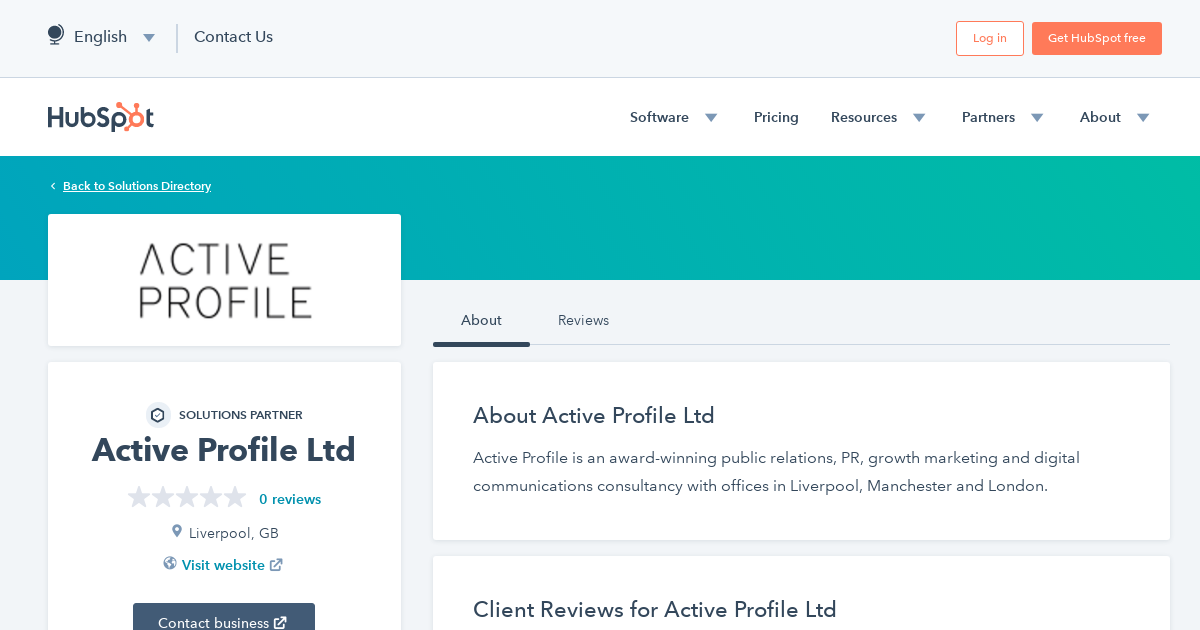At the top of the image, the header displays the text "HubSpot." On the right side of the header, there's a series of drop-down menus labeled: "Software," "Pricing," "Resources," "Partner," and "About." Each of these options expands into additional submenus. 

Beneath the header, a blue box contains a link that states "Back to Solution Directory." Below this, a white rectangular box is labeled "Active Profile."

In the main content area, there's a larger box detailing the profile of a company named "Active Profile LTD." It shows the following information: "Solution Partner," "Active Profile LTD," "0 stars," "0 reviews," and "Liverpool, GB." A blue hyperlink within this section prompts users to "Visit Website," and there's a dark blue button labeled "Contact Business."

On the right side of this section, tabs are labeled "About" and "Reviews." Underneath these tabs, there's additional information about "Active Profile LTD," describing the company as an "award-winning public relations (PR), growth marketing, and digital communication consultancy."